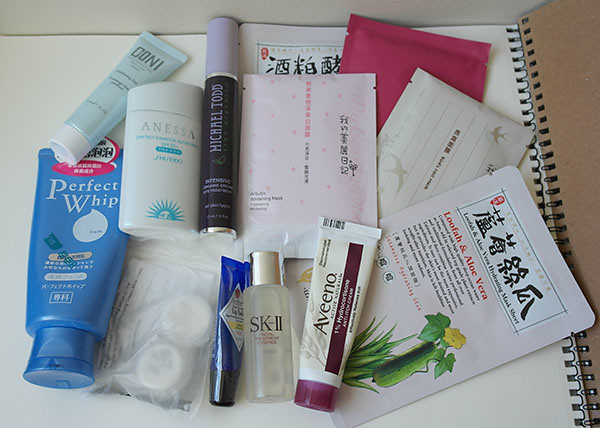This image showcases an array of toiletry and beauty products meticulously arranged on an open spiral notebook. The scene includes several items with vibrant packaging and different languages, indicating a collection of global beauty essentials.

At the center, there's a set of envelopes labeled “Luffa and Aloe Vera,” featuring Asian characters prominently on the packaging. Adjacent to these envelopes are three smaller packets also adorned with Asian writing, but their contents are not clearly visible.

To the left, a tube of Aveeno cream stands out with its distinctive white and purple color scheme. Nearby, a clear bottle labeled SK-II contains a transparent liquid, suggestive of a premium skincare product.

On the right, a blue tube of Perfect Whip facial cleanser, easily identifiable by its pop-top design, catches the eye. Next to it, there's an enigmatic plastic packet holding two white objects that could be bath beads or another form of skincare treatment.

Further to the right is a white dispenser from the ANESSA brand by Shiseido, featuring a practical pop-top. Complementing this is a small blue tube marked as "Connie," though its purpose remains unclear.

Lastly, the collection includes a striking dark purple tube from Michael Todd, distinguished by light purple writing. This diverse assortment of products rests atop a spiral-bound notebook, suggesting a well-curated and possibly travel-ready selection of beauty and toiletry items.